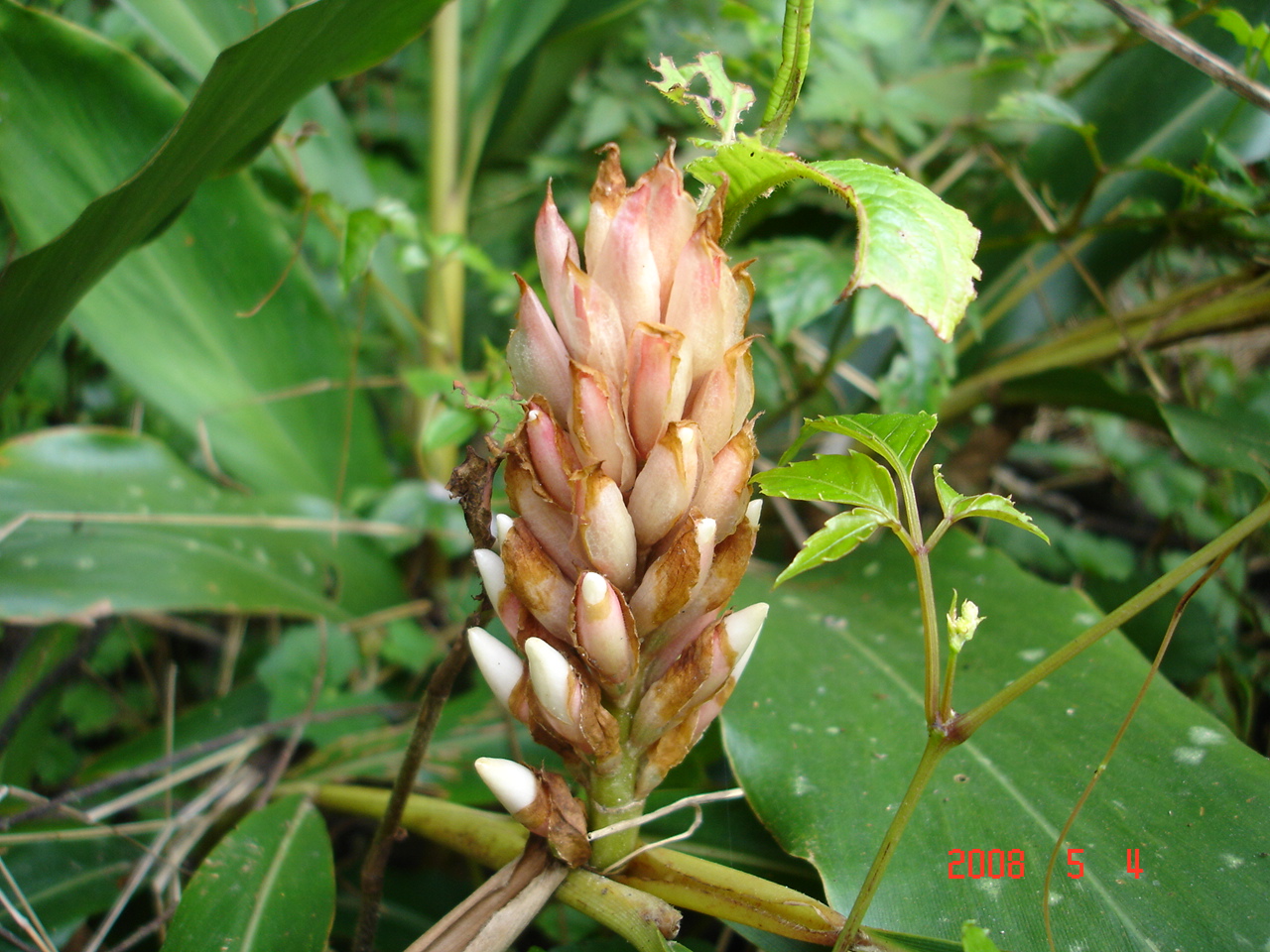The photograph showcases a close-up view of lush greenery dominated by large, banana-like leaves and abundant green stems. Central to the image is an intriguing cluster of buds emerging from one of the plants. These buds have a unique coloration, starting off white at the base and transitioning to pale pink at the tips, resembling small bananas. They appear to be in the process of blooming but haven't fully flowered yet. The buds also exhibit a peeling effect, where the brownish outer layer gives way to the lighter inner part. The surroundings are devoid of any insects, birds, or people, focusing entirely on the natural elements. Embedded in the bottom right corner of the photo is a date stamp in bright red, indicating "2008 5 4."